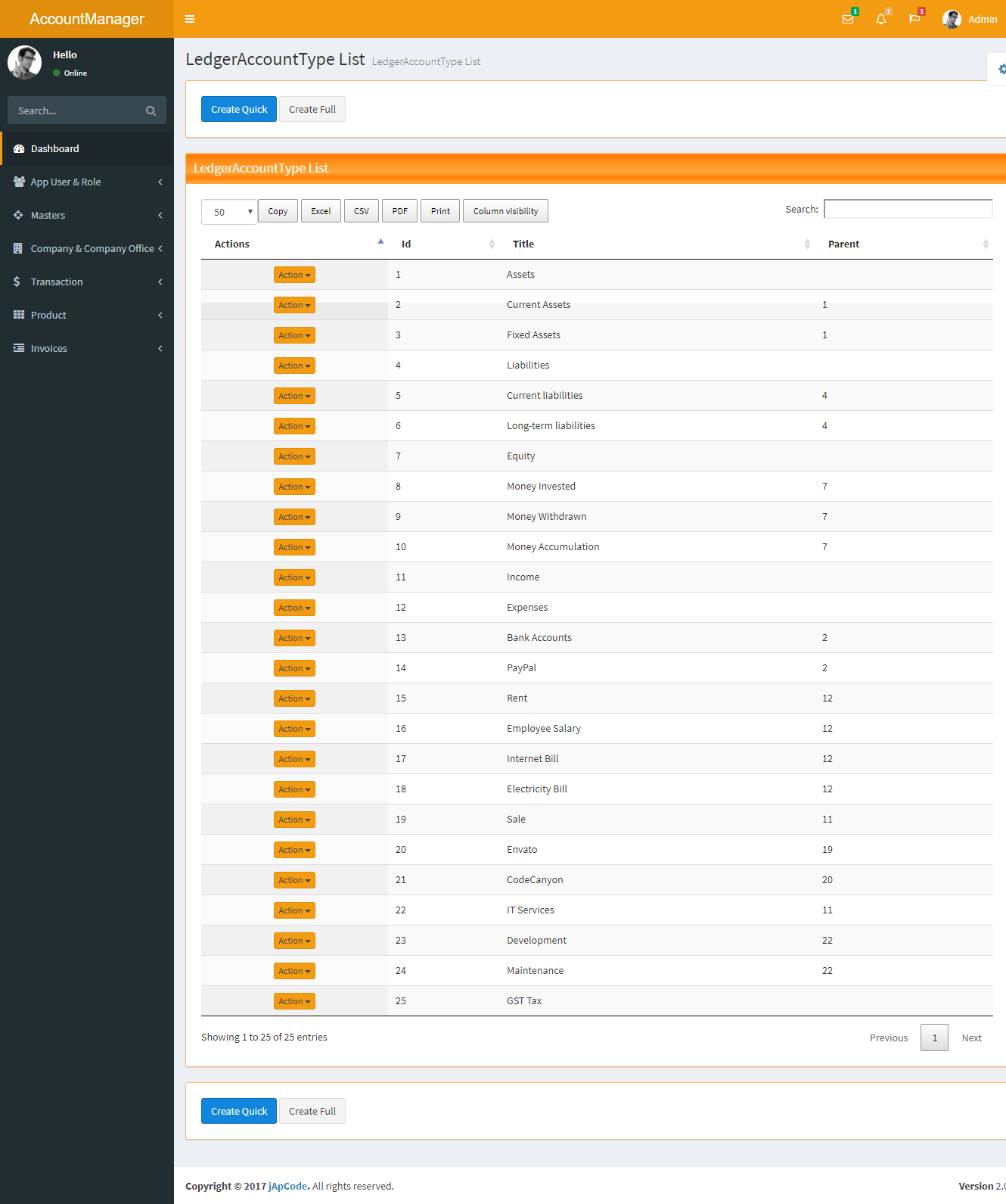Screenshot of the Account Manager Browser Interface

The screenshot displays the Account Manager's web interface. The top section of the browser is distinctly highlighted in orange. The sidebar on the left is black, featuring the user's avatar at the top—a black-and-white picture of a man. Next to the avatar, there is a greeting that reads "Hello," accompanied by a green dot indicating the user is online. Below the avatar is a search bar, followed by a detailed menu with the following items listed in sequence: Dashboard, Apps, User, Enroll, Masters, Company, Office, Transaction, Product, and Invoices.

The main section of the webpage is titled "Ledger Account Type List". Directly below this title are two buttons: "Create Quick" in blue and "Create Full". Following these buttons is a comprehensive chart titled "Ledger Account Type List", which organizes its data into four columns. Above these columns, there is a search bar on the right side, and to the left, six functional buttons: Copy, Excel, CSV, PDF, Print, and Column Visibility. Additionally, a drop-down menu set to display 50 entries is present.

The columns within the chart are labeled as Actions, ID, Title, and Parent. The Actions column contains an orange action button in each row. The ID column lists numbers sequentially from 1 to 25. The Title column includes varied entries such as "Assets" in the first row, "Fixed Assets" in the third row, "PayPal" in the 14th row, "Rent" in the 15th row, and "GST Tax" in the final 25th row. The Parent column has scattered entries, with some cells blank and others filled with numbers ranging from 1 to 22. These numbers do not follow a strict sequence, with some missing and others repeating; for instance, rows 8, 9, and 10 all have a Parent value of 7, whereas row 25 is blank.

Finally, at the bottom left corner of the chart, there is text stating "Showing 1 to 25 of 25 entries". Directly below this chart are two more buttons labeled "Create Quick" in blue and "Create Full".